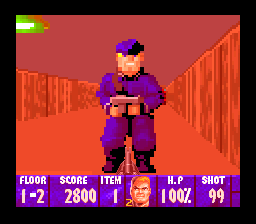In this square digital image, we're presented with a vivid scene that appears to be from a retro video game. The entire image is framed by a black border that accentuates the predominantly red hues within. The background consists of various shades of red; the ceiling is a darker red while the fencing to the right and left, as well as the ground, are lighter shades of red. 

A single, pixelated character stands out in the scene, dressed in a blue uniform and matching blue cap. The character's blocky, simplistic design gives him a Lego-like appearance, indicative of early digital graphics. Despite the low resolution, the imagery is vivid enough to provide a nostalgic charm.

At the bottom of the screen, set against a blue backdrop, white text displays crucial game statistics: "Floor 1-2," "Score 2800," "Item 1," "HP 100%," and "Shot 99." These details provide context for the game's setting and player status. Additionally, located in the center lower portion of the image, there is a square box featuring a headshot of a man. This pixelated portrait depicts him with short blonde hair and pale skin, looking directly forward, likely representing the in-game avatar or protagonist. The use of minimalist design and limited color palette effectively conveys the vintage gaming aesthetic.